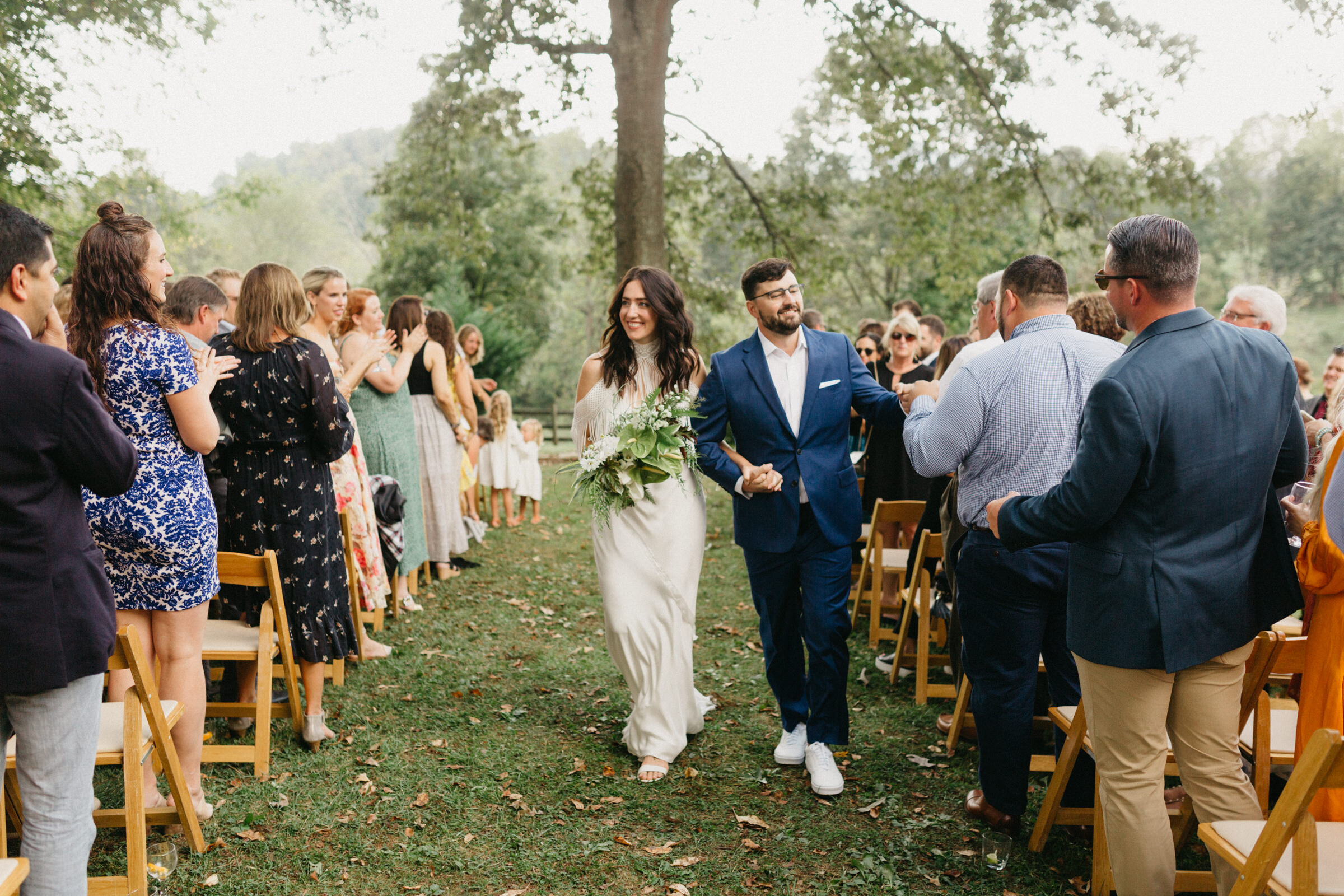This photograph captures a joyous moment at an outdoor wedding as the newlywed couple walks down the aisle amidst a standing, applauding crowd. The bride, adorned in a white dress and holding a bouquet of white flowers, has long, wavy dark hair cascading to her shoulders and is smiling gently. Her groom, a man with short brown hair, a mustache, and glasses, is dressed in a blue suit, white shirt, dark blue pants, and white shoes. Their arms are interlinked, her left with his right. 

The aisle is flanked by rows of wooden folding chairs filled with guests, who are turning towards the couple from both sides, creating a path. Some people in the distance are also turned around to witness the couple's walk. Amongst the crowd, mostly adults can be seen with a few children, likely flower girls, near the front. The scene is set on a grassy area with a few scattered leaves, under an overcast sky which evenly lights the scene. A large tree stands prominently in the middle background, with green hills and forested areas visible in the distance, suggesting a setting in a hilly or mountainous region.